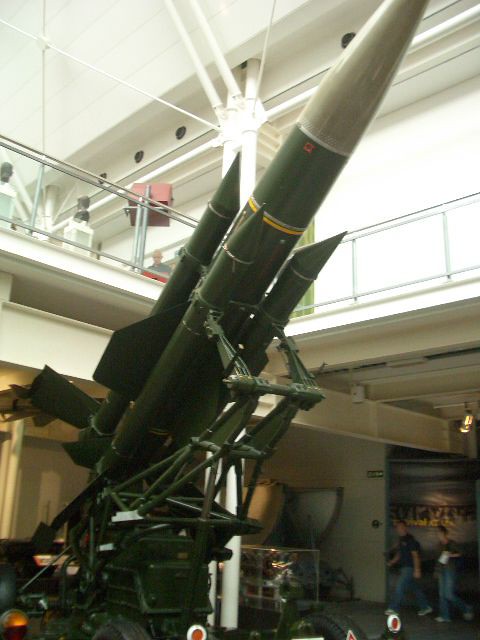The photograph captures an impressive scene of a rocket launch exhibit at what appears to be a museum. This enormous rocket, with its base mounted on a specialized launcher, extends beyond the second story of the building, highlighting its monumental size. The rocket features a partially army green body with a gray tip, suggesting a historical or military design. On the ground floor, two individuals can be seen walking, while a solitary observer stands on the upper level, gazing up at the towering rocket. Adjacent to the rocket, there is another indistinct object, adding an element of intrigue to the scene. The overall composition of the photo not only showcases the rocket's grandeur but also provides a glimpse into the museum's multi-story layout and the curiosity it sparks among its visitors.